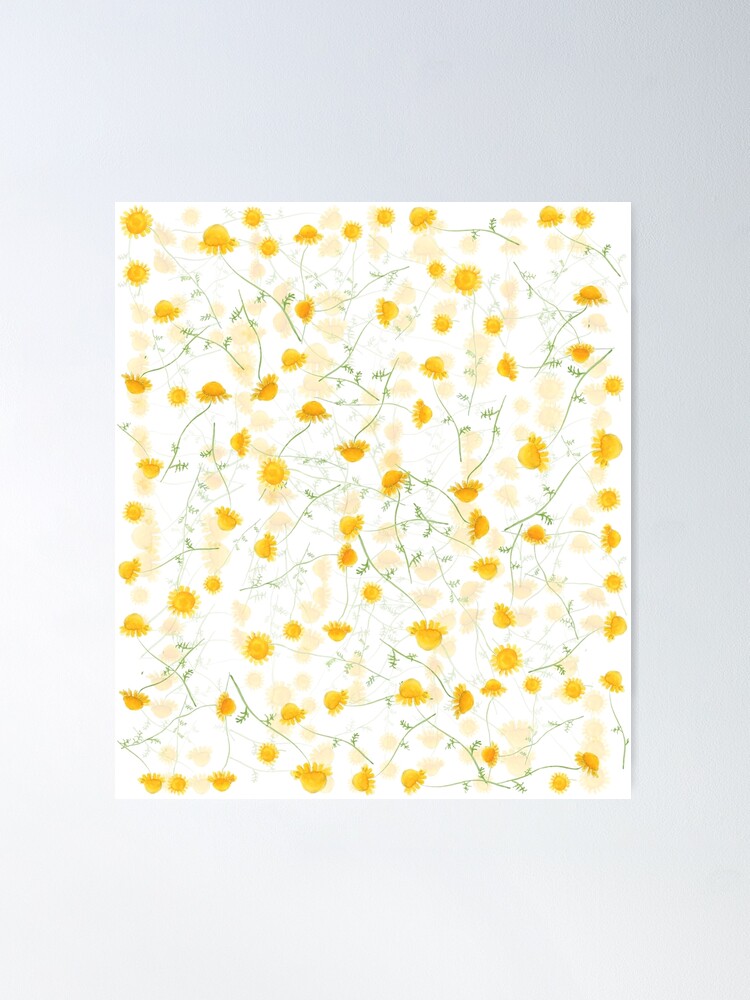This photograph captures a detailed painting mounted on a light gray wall. The painting itself, on a frameless white canvas, prominently features numerous delicate yellow flowers resembling dandelions or daisies. Each flower has a circular head adorned with many tiny yellow petals and is attached to a thin green stem with occasional small leaves. The flowers are assorted randomly, facing different directions—upward, downward, left, and right—creating an intriguing pattern that covers the entire canvas. The overall background of the painting has a white or ivory tone with subtle hints of pinkish shading. Interspersed among the clear golden flowers are paler, semi-transparent ones, adding depth and texture to the artwork. The combination of crisp and faded flowers along with the greenish-gray stems and a sprinkling of scattered green leaves brings a lively yet harmonious appearance to the piece, reminiscent of a meticulously crafted wallpaper design.